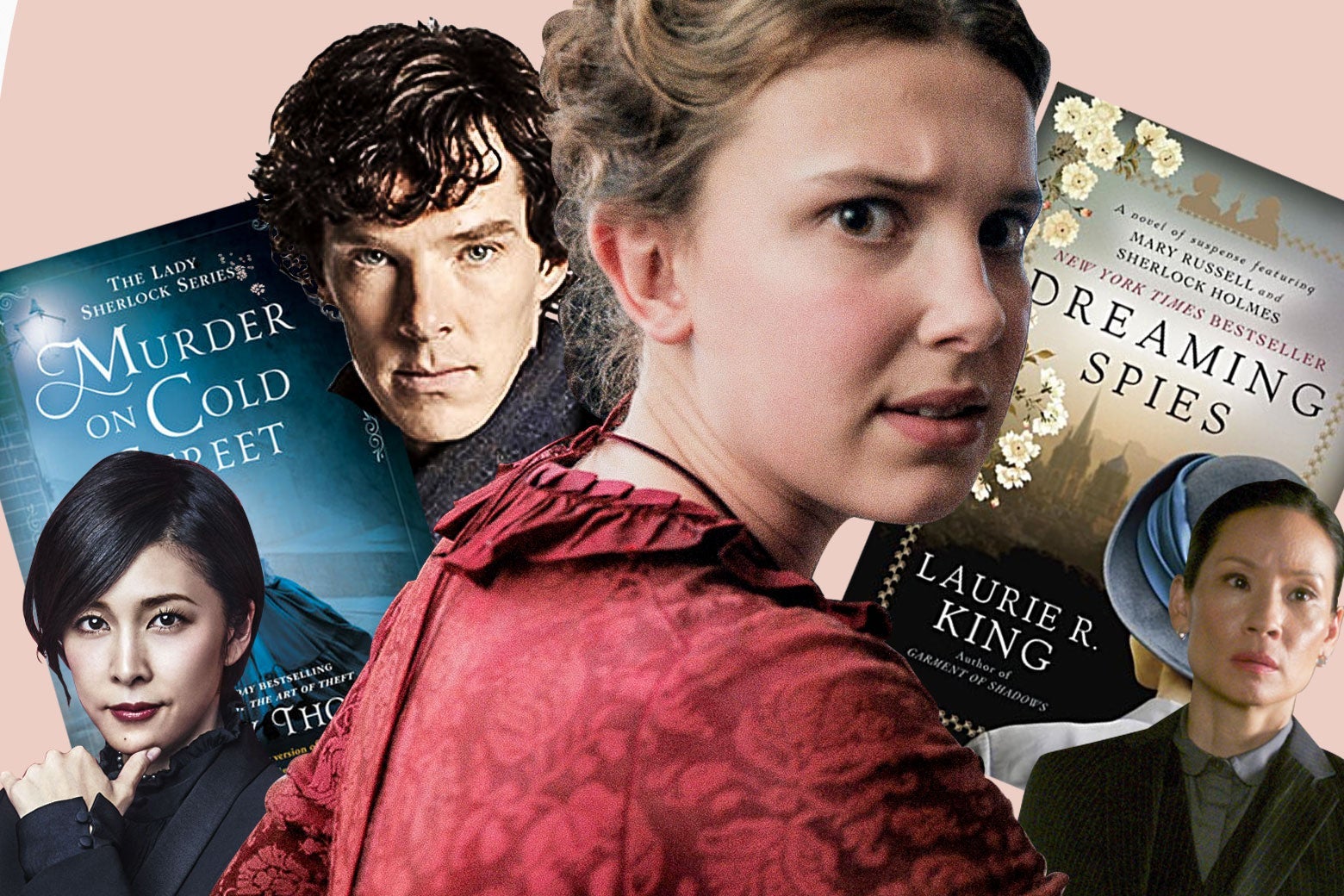This is a composite image featuring a combination of well-known actors and book covers related to the Sherlock Holmes universe. Central to the image is Millie Bobby Brown, known for her role as Enola Holmes on Netflix, adorned in a deep red brocade dress with her hair elegantly pulled back. Positioned behind her are Benedict Cumberbatch, who portrays Sherlock Holmes in the series "Sherlock," and Lucy Liu, recognizable from her role in "Elementary." The background further features another actress whose name is not immediately known. The entire setup is placed against a pink background with visible book covers interspersed. These book covers include "Dreaming Spies" by Laurie R. King, prominently displayed, and "Murder on Cold Street" from the Lady Sherlock series, although the author’s name is obscured by another actress in the foreground. The image focuses primarily on the characters' faces, creating a visually engaging montage that connects the actors through their association with Sherlock Holmes stories.